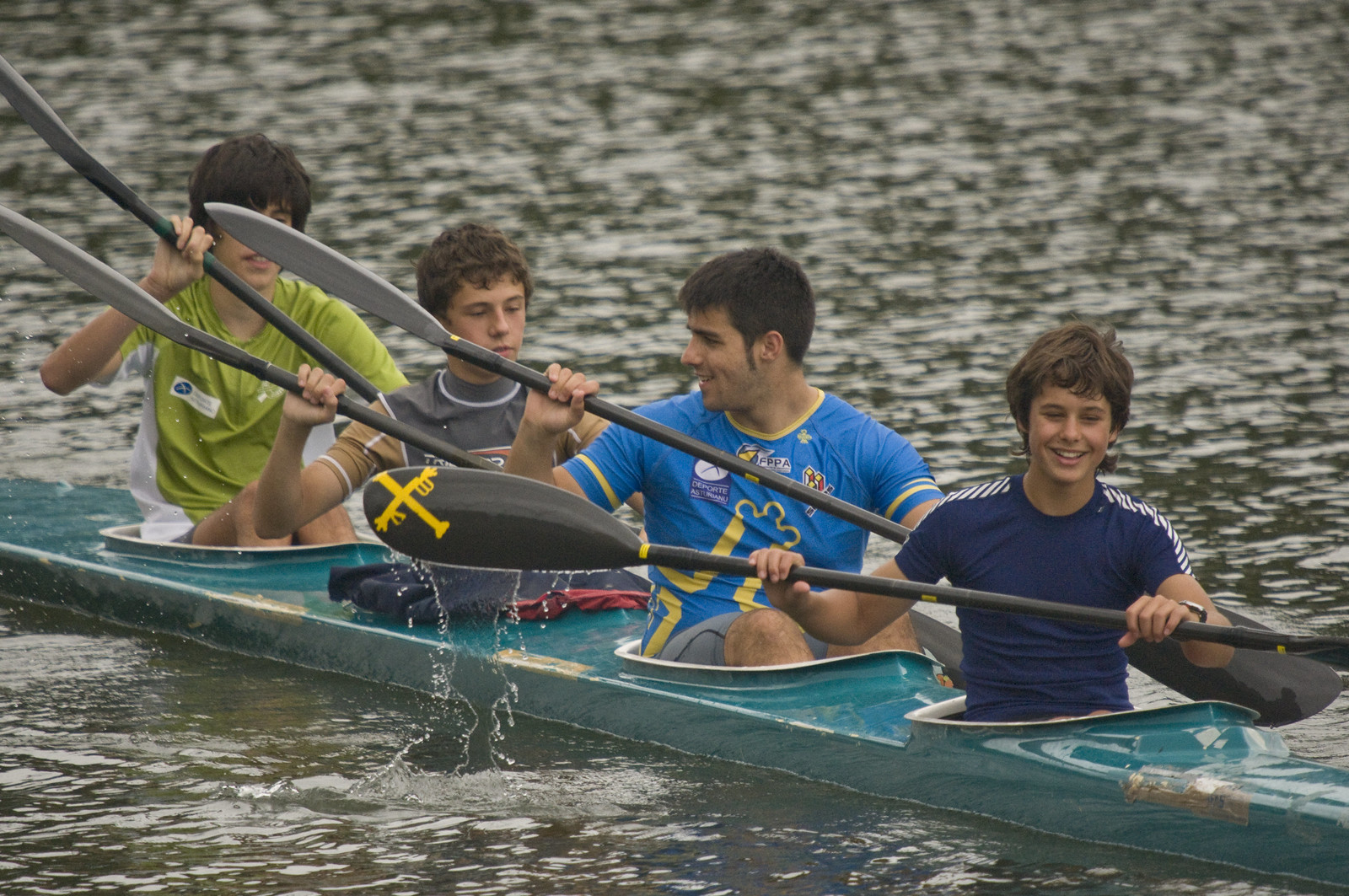This image depicts four young men seated in a four-person, shiny medium-blue crew boat on a body of water, possibly a lake or river. The crew, ranging in age from around 15 to the early twenties, each hold a double-sided paddle. The young man at the back, wearing a green shirt, is observed paddling with one side of his oar, which has gray and black colors, while a second visible paddle features a yellow cross. In front of him sits a boy in a gray short-sleeve shirt, followed by another in a blue short-sleeve jersey with yellow details. Leading the group is a boy in a dark-blue jersey with distinctive white shoulder stripes. They navigate the black water in what appears to be a casual or training session rather than a competitive event, and all seem to be enjoying their time on the water. The boat is partially visible and might have more seats, but only these four paddlers can be seen in the image.